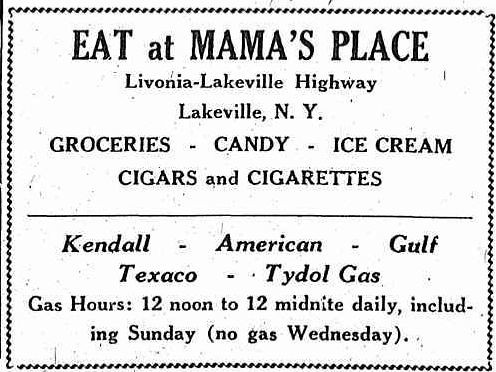This black-and-white advertisement, with a smudgy, low-quality appearance reminiscent of an old newspaper or magazine ad from 40-50 years ago, is split into two sections by a horizontal black line with a zigzag outline surrounding the entire border. The top section promotes "Eat at Mama's Place" located on Livonia Lakeville Highway, Lakeville, New York, offering groceries, candy, ice cream, cigars, and cigarettes. The bottom section lists gas stations, indicating "Kendall-American-Gulf" and "Texaco-Tidal Gas". The gas hours are 12 noon to 12 midnight daily, including Sundays, with a note in parentheses specifying "no gas Wednesday." The advertisement is slightly wider than it is tall but nearly square, with very basic and unattractive font.